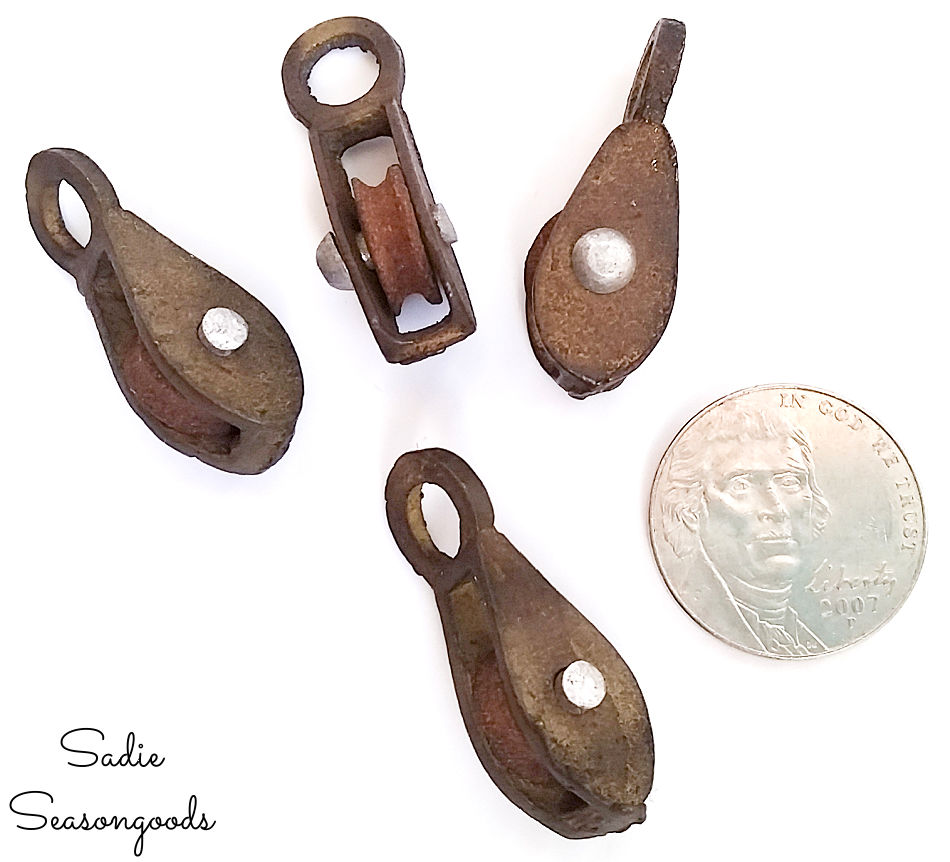This close-up photograph features four rusted pulley mechanisms, each displaying significant wear with a mix of dark and light brown rust. These mechanisms are showcased on a stark white background, emphasizing their aged texture and intricate design. Each pulley has a central wheel encased in a rusted housing, connected by a rivet or bolt that allows the wheel to turn freely. Notably, these pulleys are positioned at various angles to reveal different sides and functional details, including an eye loop set at a 90-degree angle from the wheel.

A Jefferson nickel, in silver color, is strategically placed in the image to indicate the size of the pulleys. The nickel displays the head of Thomas Jefferson with the inscriptions "IN GOD WE TRUST," "LIBERTY," and the year "2007," along with a visible mint mark. The attention to detail extends to the nickel, highlighting its intricate design. In the bottom left corner of the image, the text "Sadie Season Goods" is written in black script, adding a subtle branding element to the photograph.